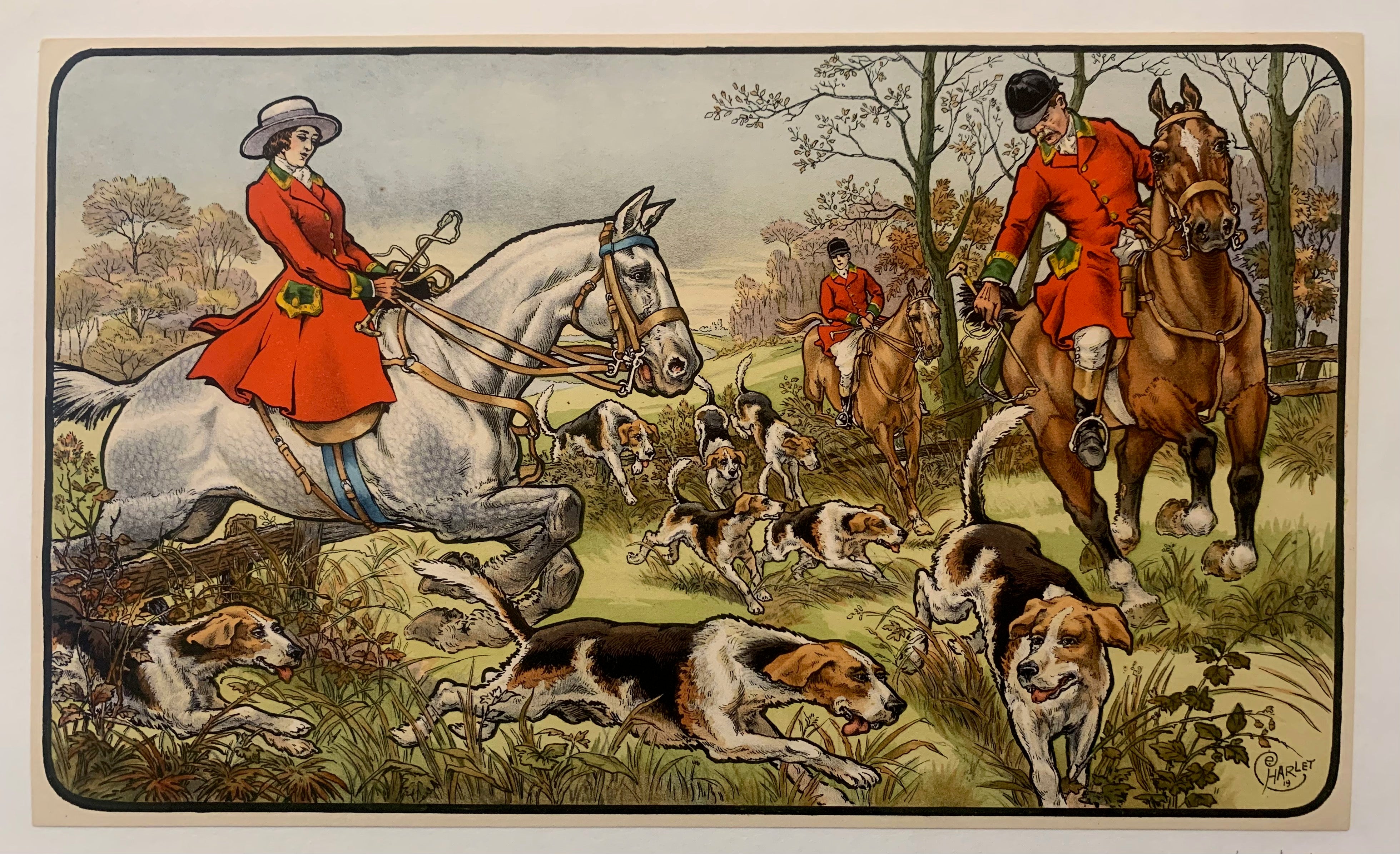This vintage artwork, resting on a white table, is a signed piece by Harlett, evident from the signature in the lower right corner. The illustration depicts an outdoor scene reminiscent of the English countryside, possibly from the 1800s or early 1900s. The colors are muted, giving it an aged, antique appearance. The setting features three riders in red jackets: a woman atop a white horse, wearing a brimmed white hat and sitting side-saddle, and two men on brown horses, both donning black hats. They are accompanied by a pack of six to seven hunting dogs, primarily beagle-like in their white, black, and brown coats. The dogs run energetically across a verdant green pasture dotted with various plants, fences, and distant trees, likely in pursuit of a hunt. In the background, rolling hills enhance the pastoral charm of this historical scene.